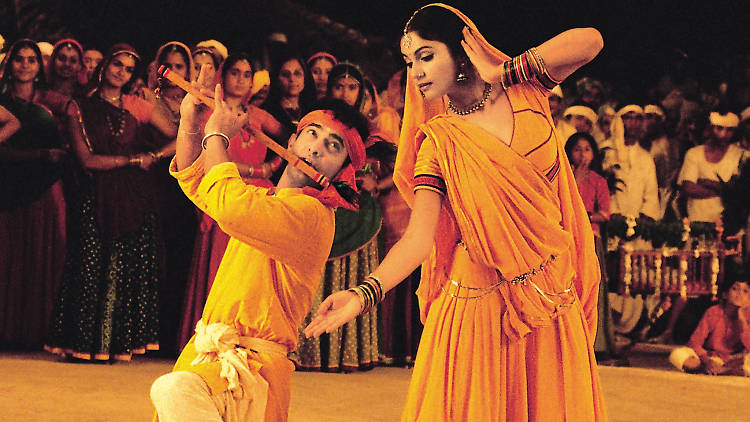In the image, there is a vibrant scene featuring two individuals, likely from India, based on their traditional attire. The woman in the foreground is draped in a flowing orange dress and has a shawl covering her head. She is adorned with multiple rings on her arms, a necklace, and a delicate nose ring. She is depicted with one hand placed gently on the side of her head and the other extended downward. Next to her is a man dressed in matching orange clothing, equipped with a red band tied around his forehead. He is kneeling and looking up at the woman while playing a yellow flute-like instrument. The background reveals a large crowd, all dressed in similar traditional attire, observing the duo. The scene takes place on a yellow-tiled floor, and there is an indistinct device located at the bottom right corner of the image. The overall atmosphere is rich, celebratory, and culturally immersive.